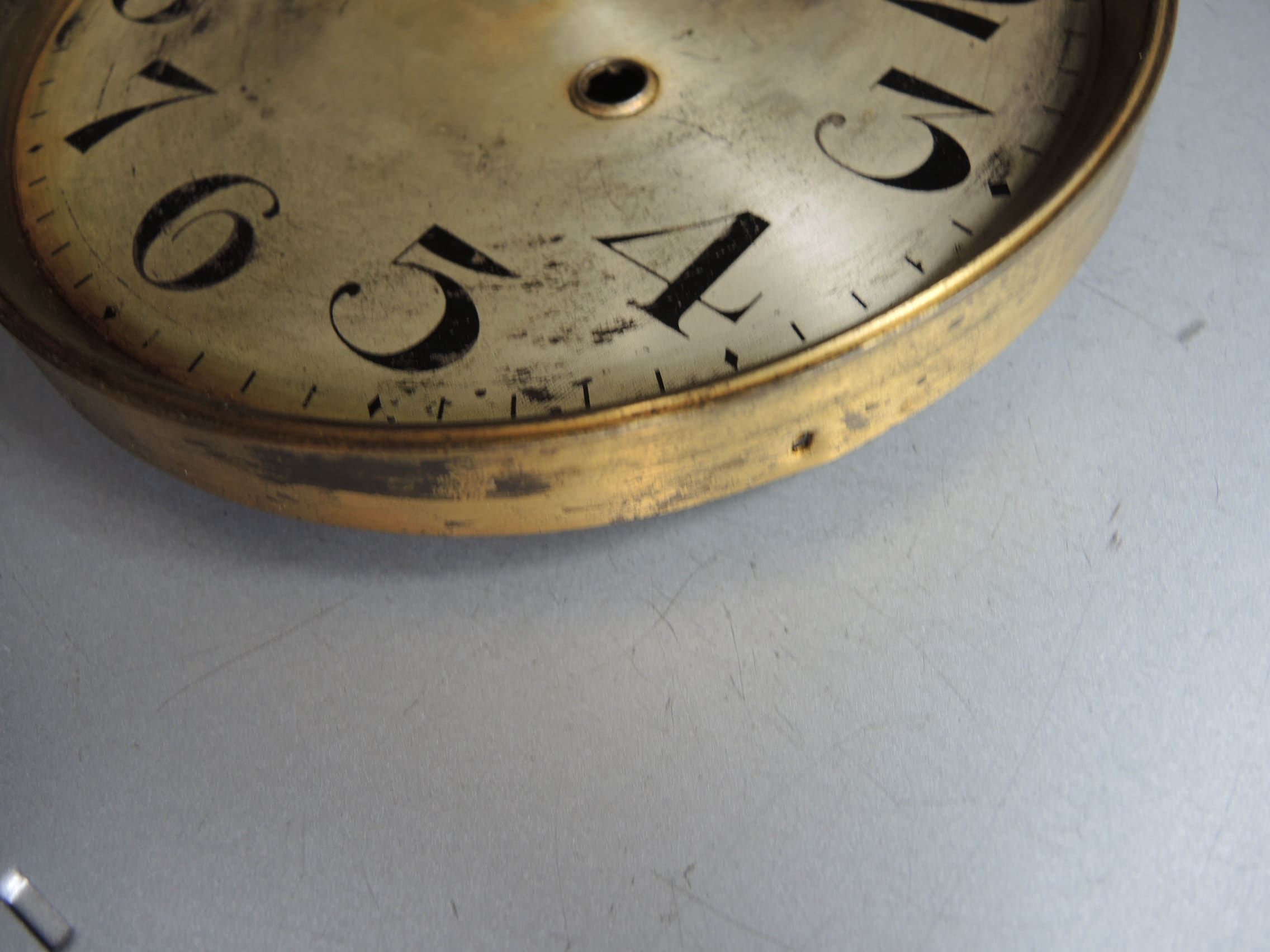The photograph is a staged, square, full-color image taken indoors with artificial lighting. The background is a bluish, scuffed table or countertop that appears brighter in the lower right corner and darker in the upper left. The lower left corner of the image reveals a piece of indistinguishable silver material. Dominating the upper left to the right-hand side is a prominently featured old clock face with a tarnished brass or gold rim, showing significant signs of wear, including black spots, holes, and patches. The clock face is a very aged white or light yellow-tan, also marked with black scuffs and scratches, indicative of its vintage condition. The visible black numbers on the clock are 3, 4, 5, 6, 7, and part of the bottom of 8. In the center of the clock face, between the 3 and 4, there is a circular indent with a light gold ring around it, likely where a key would be inserted to wind the clock. The clock lacks visible hands, adding to its worn, antique appearance.